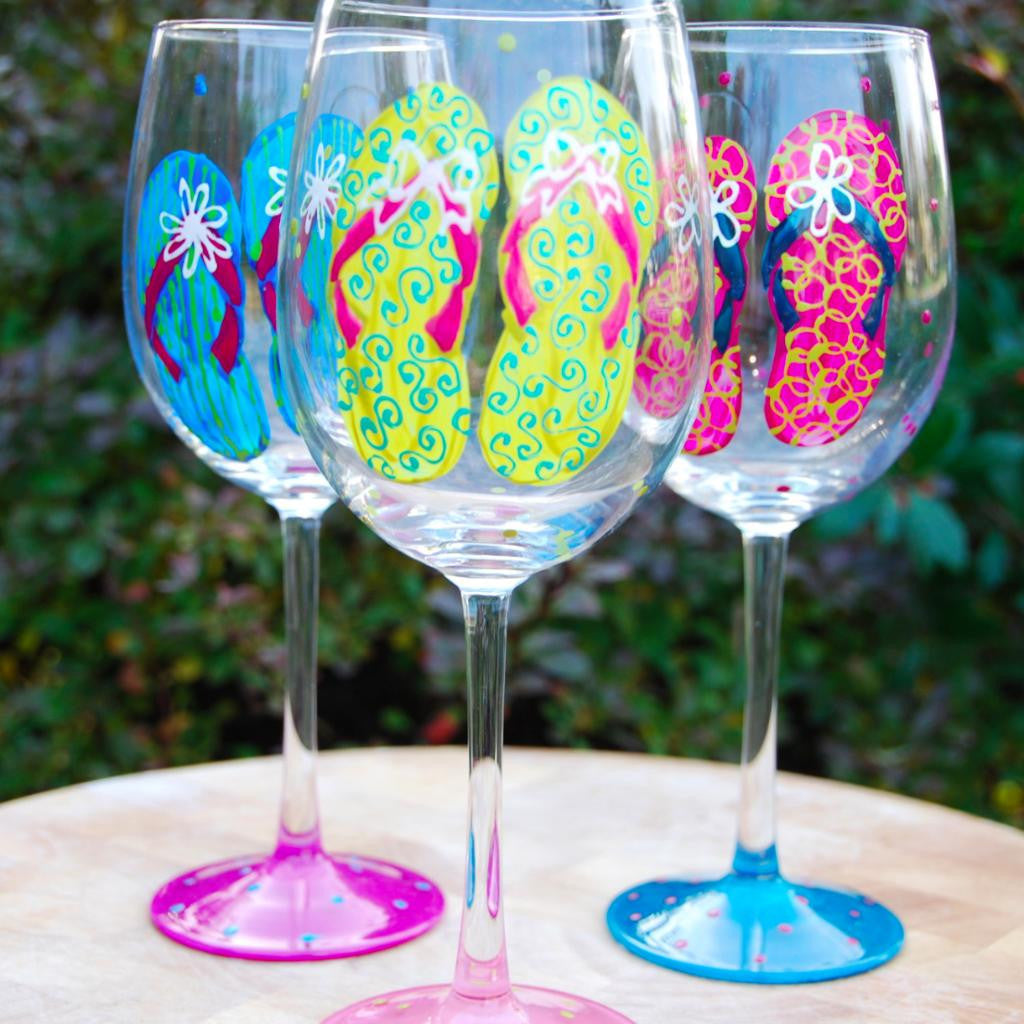The image features three uniquely designed wine glasses standing on a circular table. The background is predominantly filled with dark green hues and a variety of plants, which occupy the top three-fourths of the scene. 

The glasses, each with unique artistic details, are positioned strategically: the one closest to the viewer, whose bottom is partially cropped out of the image, is light pink with yellow dots. It features yellow painted sandals adorned with purple straps and white bow strings, with an intricate design of fancy "S" shapes decorating the sandals. The glass on the back left is dark purple with blue speckles. It showcases blue flip-flops with red straps and eight flower petals surrounding it. Lastly, the glass on the right, which displays a blue hue with pink dots at its base, is decorated with purple flip-flops, black straps, and a five-leaf clover flower design.

Bringing together the individual details and common elements, the composition presents a vibrant and intricate still-life scene with a whimsical touch of custom-designed flip-flops accentuating each wine glass.